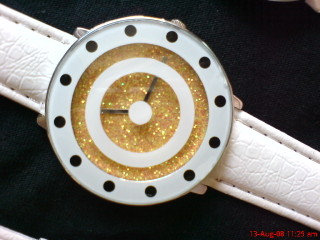This close-up image showcases an elegant white watch set against a sleek black background. The watch features a white leather band adorned with precise stitching along both sides, exuding a sense of refined craftsmanship. The watch's face is intricately designed, presenting a unique, almost target-like pattern. At the very center, a pristine white dot captures attention, encircled by a slender band of glittering gold. Surrounding this, a wider white circle further enhances the design, which is highlighted by a ring of minimalist black dots in place of traditional numbers. Each dot is meticulously placed to denote the hours. The sleek black hands of the watch point to approximately five minutes past 10. The watch face is accentuated by a background of shimmering gold, adding a touch of luxury. Subtle numbers and letters are visible on the lower right-hand side of the watch face, though they remain difficult to decipher.